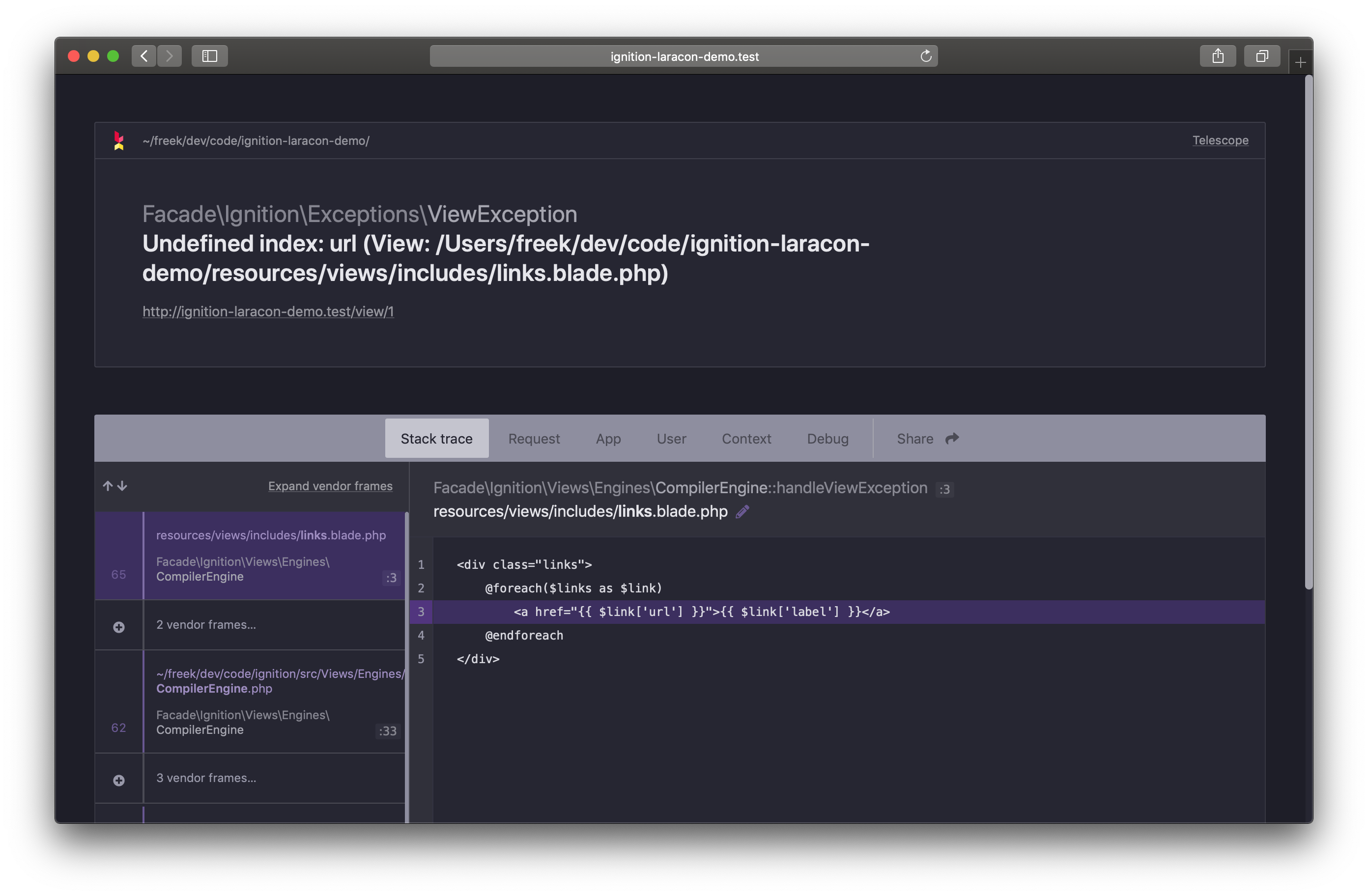This image depicts a MacBook screen displaying a webpage with the URL "ignition-laracon-demo.test" visible in the browser's address bar. The page is showcasing an error message featuring a summary of a coding issue. The error mentions a "FACADE" issue related to "ignition", specifically pointing to an "undefined index" in the "column" parameter within the following file path: "/users/freq/dev/code/ignition-laracon-demo/resources/views/includes/links-blit.php". The error details are encapsulated within a framework path format, hinting that this could be a part of a larger stack trace.

The webpage features a black and blue color scheme, providing a high-contrast backdrop for the error message and various debug information. Notable keywords displayed include "stack trace," "request," "app," "user," "context," "debug," and "share," suggesting sections dedicated to troubleshooting and debugging the error. Towards the bottom of the page, there is a small segment containing five lines of code, which likely relates to the error context. This detailed error display indicates that the page is part of a developer tool or environment aimed at diagnosing and resolving code issues efficiently.